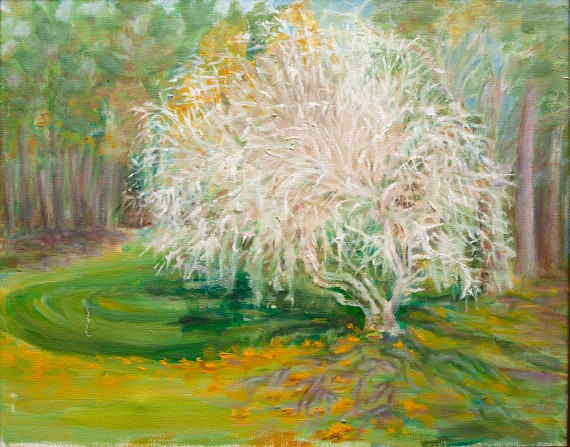This is a vibrant and detailed painting of a forest scene dominated by a large white willow tree in the foreground. The painting features an array of greens and yellows, with touches of white and brown. The background depicts several tall trees with green and yellow leaves atop light brown trunks, creating a dense forest backdrop. The ground is a mix of green and yellow hues, with some specks resembling flowers and a conspicuous green blotch that suggests a pond covered in algae. The central focus is the imposing white willow tree, which has a prominent trunk that branches out in the middle. Its long branches are bare, lacking leaves, allowing the intricate details of the white branches to stand out. The roots of the tree extend into the brownish soil. This colorful artwork, possibly done in chalk, highlights both dark and light green shades with yellow accents, creating a dynamic and bright composition. The overall scene is enhanced by the veining of the willow's roots painted onto the ground and the presence of shaded brown areas, contributing to the depth and richness of the image.